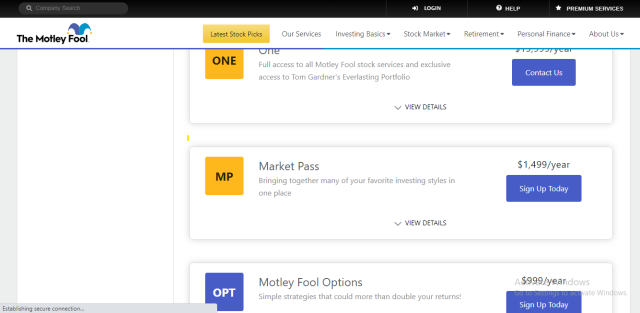The image depicts a screenshot of a computer webpage with a predominantly white background. A black bar stretches across the top of the page, featuring a slightly lighter-colored search bar on the left side and three white-lettered words on the right. Below this, a white bar spans the width of the page, marked with a blue underline. The text "The Motley Fool" appears here, accompanied by a graphic of a jester's cap above the word "Fool."

To the right of this, a noticeable yellow button provides some call-to-action text, and six clickable words suggest the presence of a dropdown menu. Moving further down, the main section of the screen shows a largely blank white area on the left, with three horizontally aligned white rectangles. The first and third rectangles are partially obscured at their top and bottom edges, respectively. The top and middle rectangles each feature an orange square on the left; the top one has the number "1," and the middle one is marked with "MP."

Each rectangle contains a title in a darker font, followed by a brief descriptive sentence underneath. A downward-facing caret suggests more information is available under "View Details." The bottom two rectangles also contain a blue square button with options such as "Contact Us" or "Sign Up Today."